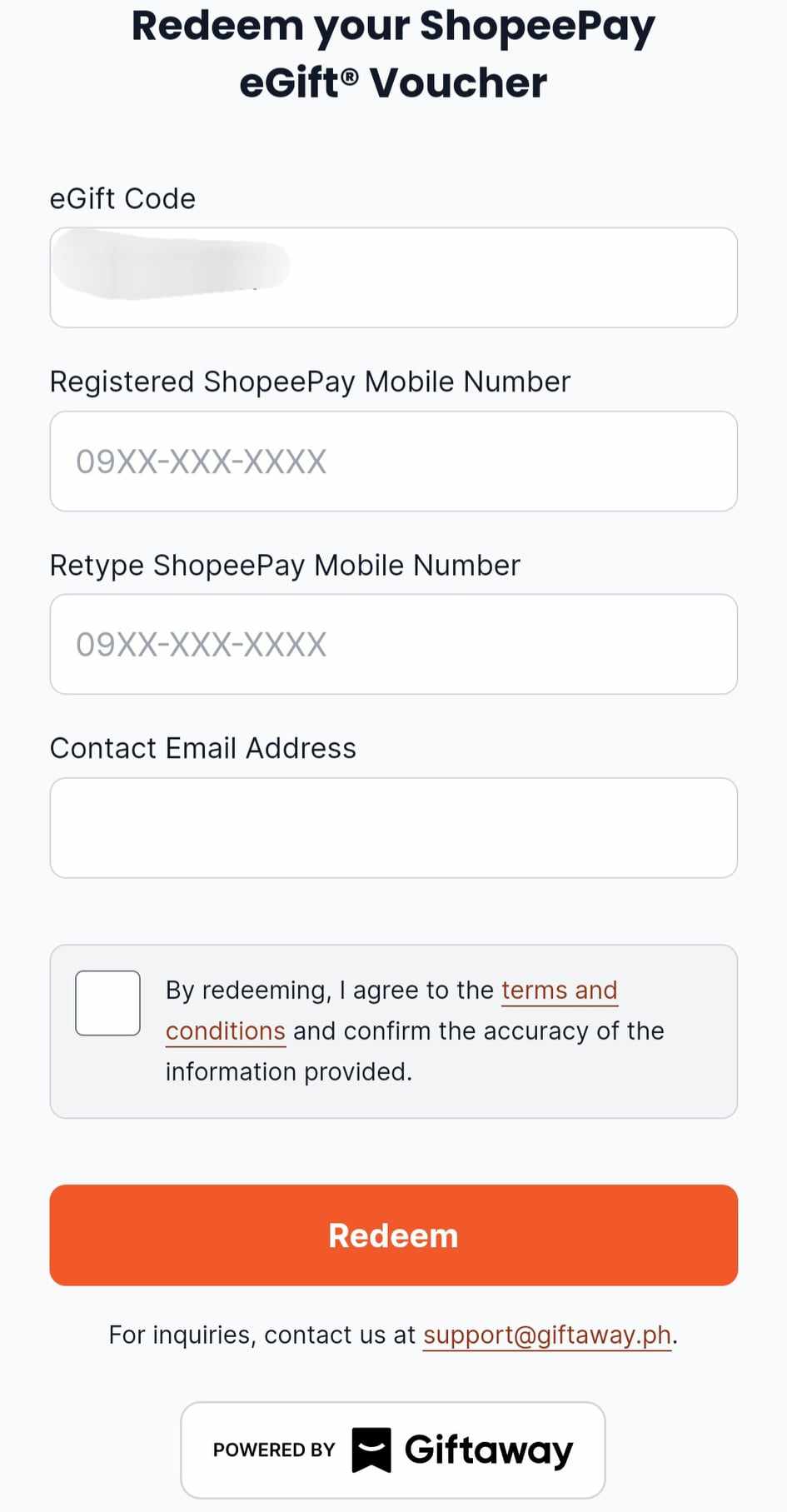This image provides a step-by-step guide for redeeming your ShopPay e-gift voucher against a light gray backdrop. Central to the image are several form fields and instructions. Starting from the top, there's a white box for entering your e-gift code, with previous information whited out for privacy. Below this are two white boxes: one for your registered ShopPay mobile number and another for retyping it for confirmation. Following these, there's a field for entering your contact email address.

Adjacent to these form fields, there is a small checkbox labeled "By redeeming, I agree to the terms and conditions and confirm the accuracy of the information provided," which must be checked to proceed. Below the checkbox, an orange 'Redeem' button is prominently displayed, with the word 'Redeem' in white letters.

At the bottom of the image, in red, clickable, underlined text, it reads, "For inquiries, contact us at support@giftaway.ph." This offers a point of contact for users needing assistance. The image also notes that the service is powered by GiftAway, featuring a black ribbon with a white smiley icon within a white box.